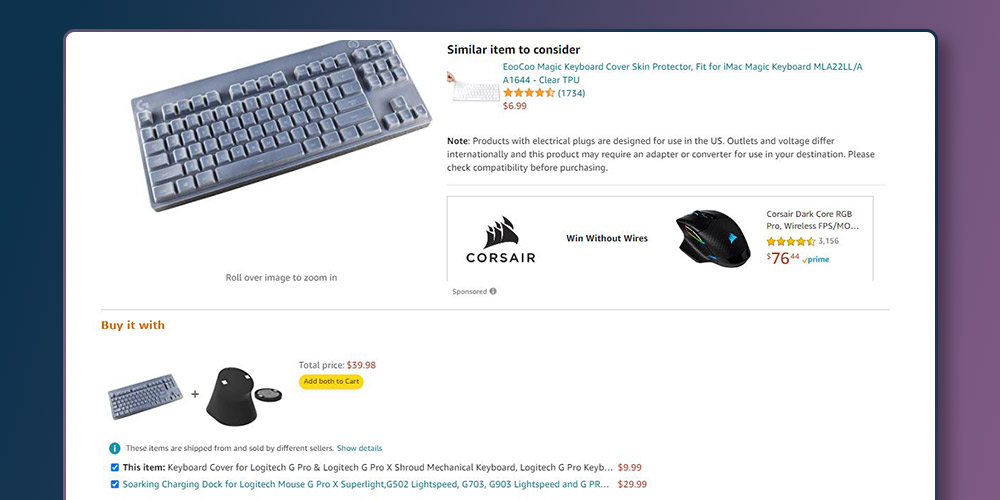This image is a screenshot of an Amazon product page featuring a Logitech keyboard. The layout is a familiar Amazon format, identified by the "Buy it with" section at the bottom of the page. This section displays a keyboard at the top, with an additional related device shown below it, linked by a plus sign. The total price for both items is listed as $39.98 in red text. Below the price is a yellow "Add both to cart" button. Two checked boxes indicate the selected items: 

1. A keyboard cover for Logitech G Pro and Logitech G Pro X Shroud Mechanical Keyboard, priced at $9.99.
2. A Sorkin charging dock for Logitech Superlight Lightspeed G703, priced at $29.99 in red text.

At the top of the page, there is an image of a gray keyboard with a traditional layout, including F1 through F12 keys, the Escape key, and the number row. 

To the right, a sidebar labeled "Similar item to consider" features a white keyboard and an Eco Magic Keyboard Cover Skin Protector priced at $6.99. 

Additionally, there is a note about products with electric plugs being designed for US outlets. Featured lower down on the page is a Corsair logo, with options for products with or without wires. Also showcased is an expensive Corsair Dark Core mouse, complete with reviews and a price of $76.44.